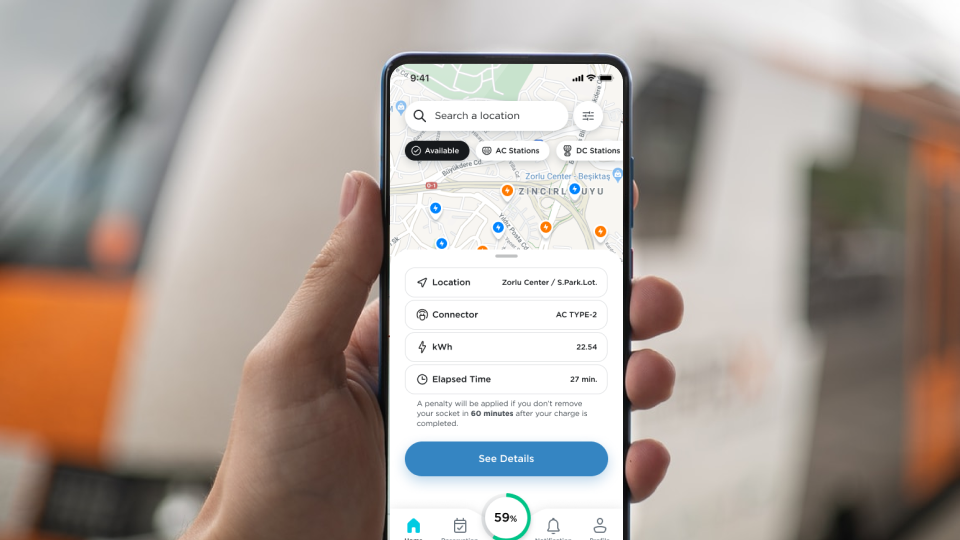The photograph prominently features a close-up of a Caucasian person's left hand holding an iPhone against a blurred background. The iPhone's screen displays a map application, highlighted by the clear visibility of the battery, cell signal, and wireless connection icons in the top corners of the screen. The time reads 9:41 in the top left corner.

The map screen in the foreground includes a search text box labeled "Search a location" at the top. Below this are three selectable options: "Available," "AC stations," and "DC stations." The map itself is marked with various pins. Among them, four blue pins with lightning bolt symbols and two blue pins with briefcase-like symbols can be noticed. Additionally, a few pins with orange centers and lightning bolt symbols are evident on the map. 

The map features text labels marking specific locations such as "Zorlu Center" and "Beşiktaş" along with various street names, indicating it is a city map. 

At the bottom of the map screen, location details are provided: "Zorlu Center South Parking Lot Connector AC Type 2," with specifications reading "KWH 22.54," and an "Elapsed time of 27 minutes."

The photograph is set against a highly blurred background, where a possible white vehicle and some orange elements can be faintly discerned, but remain indistinguishable.